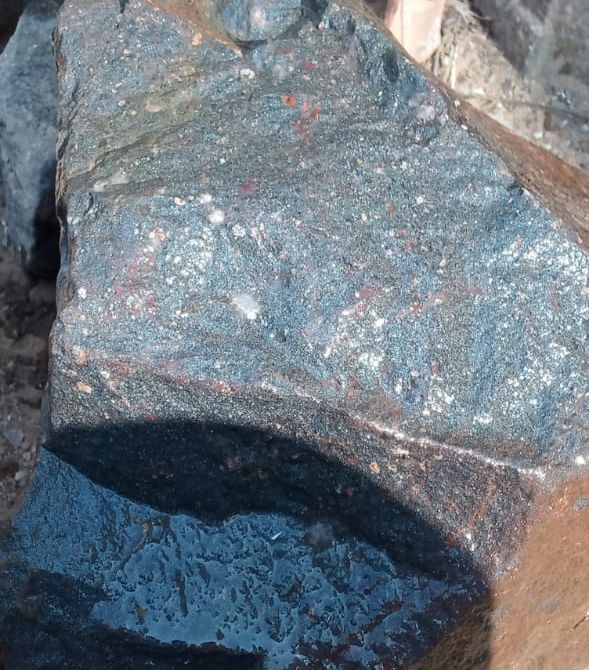This highly detailed close-up photograph captures a rugged, angular dark gray rock as the central focus, illuminated by bright daylight. The rock’s texture is accentuated by various specks and flecks, including white, reddish-pink, and rust-colored accents. The lower portion of the rock shows signs of moisture, appearing shinier and slightly wet, with a darker shadow hinting at the rock's uneven surface and the sunlight's intense illumination. Surrounding the main rock, additional stones of varying gray shades, some light and some matching the gray of the central rock, can be seen. The bottom right corner features a patch of dark brown mud or clay, adding to the natural, earthy setting.